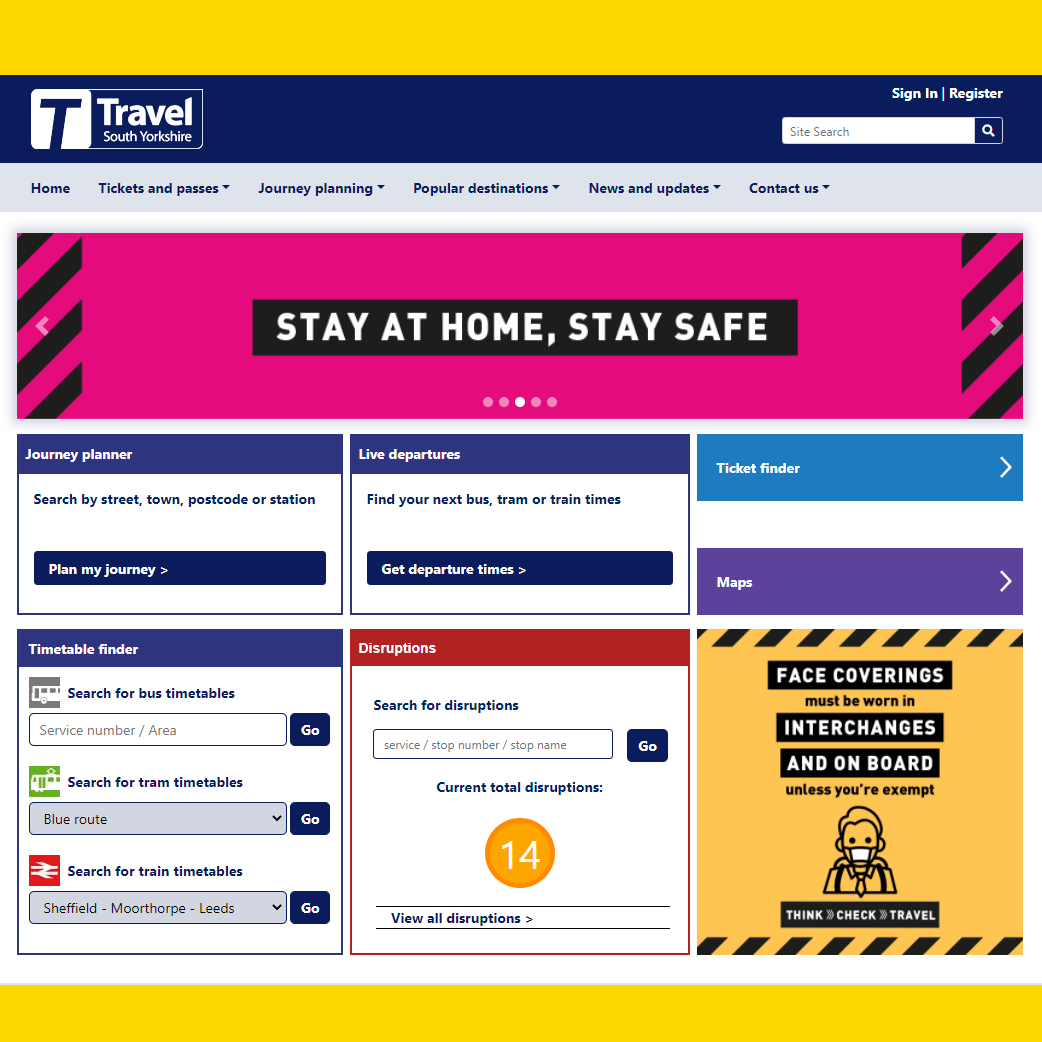This image is a detailed screenshot of the "Travel South Yorkshire" website. The design of the page features yellow bars at both the very top and bottom. Directly beneath the top yellow bar is a dark blue bar, prominently displaying the website's logo on the left side. The logo consists of the text "Travel South Yorkshire" and a solid white square with a dark blue 'T’ icon to its left. On the right side of this blue bar, a search bar is positioned for user convenience.

Beneath the blue bar is the primary navigation menu, which contains six clearly labeled buttons: "Home," "Tickets and Passes," "Journey Planning," "Popular Destinations," "News and Updates," and "Contact Us." This menu is followed by a slider module featuring a visually striking pink and black graphic. In the middle of this graphic, a black bar displays the message "Stay at Home, Stay Safe" in white text.

Further down the page, the layout transitions into a three-column structure comprising six distinct sections, with two sections neatly organized within each column.